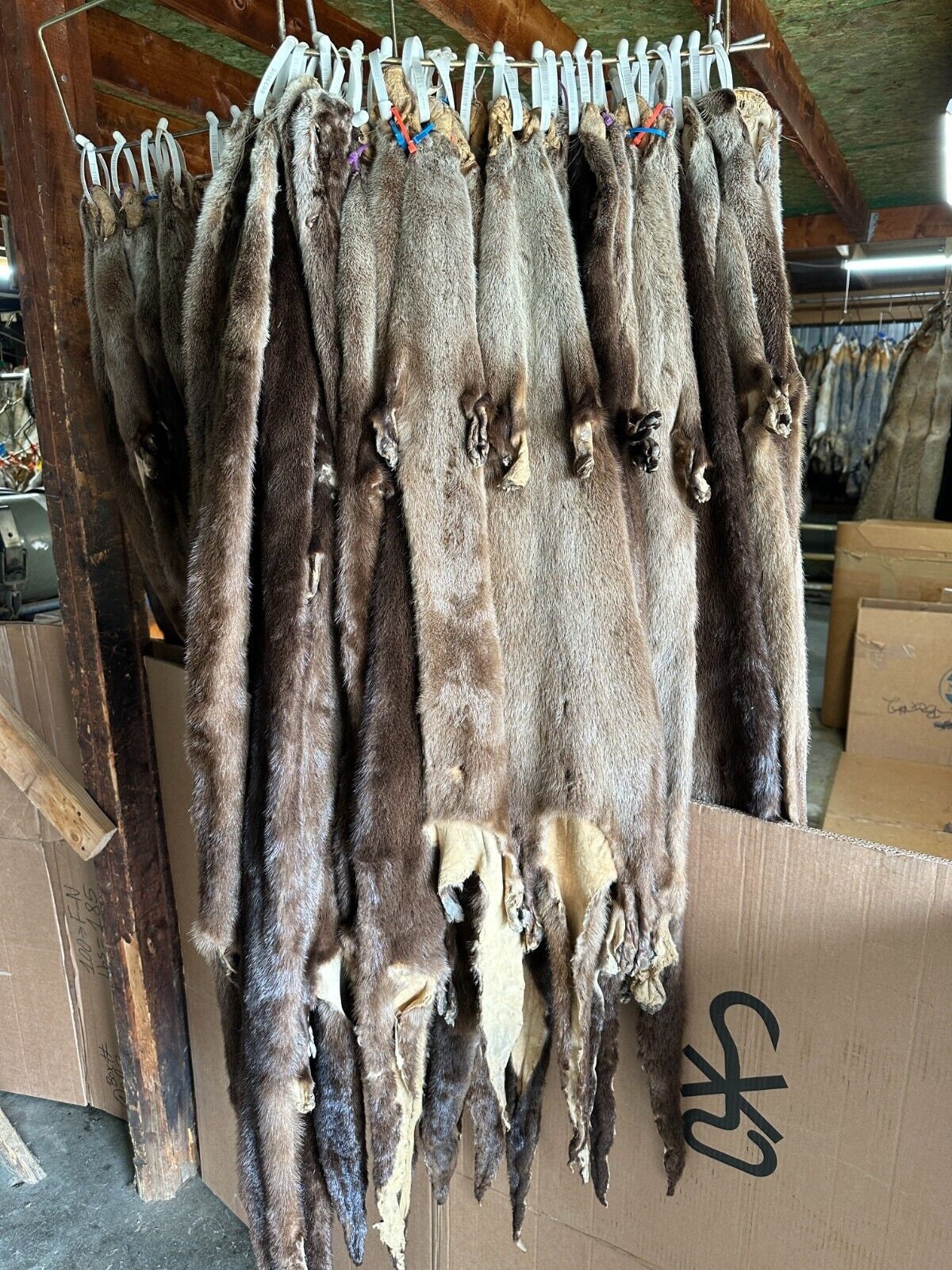This image reveals a seemingly unsettling scene set in an outdoor market, likely located outside of the United States. The focal point is an array of animal pelts, predominantly seal skins, displayed prominently. These pelts are hung from a beige clothesline using white clips, creating a grim visual with their flattened forms and visible flippers. The foreground features two hooks densely laden with these pelts, suggesting a significant quantity, with estimates ranging from a dozen to possibly forty. The backdrop, cluttered with cardboard and wood beams, hints at additional sections where more pelts or potentially coats are displayed. The setting, although appearing to be outdoors, has elements like wood paneling and an unfinished-looking ceiling, contributing to the overall disconcerting atmosphere.